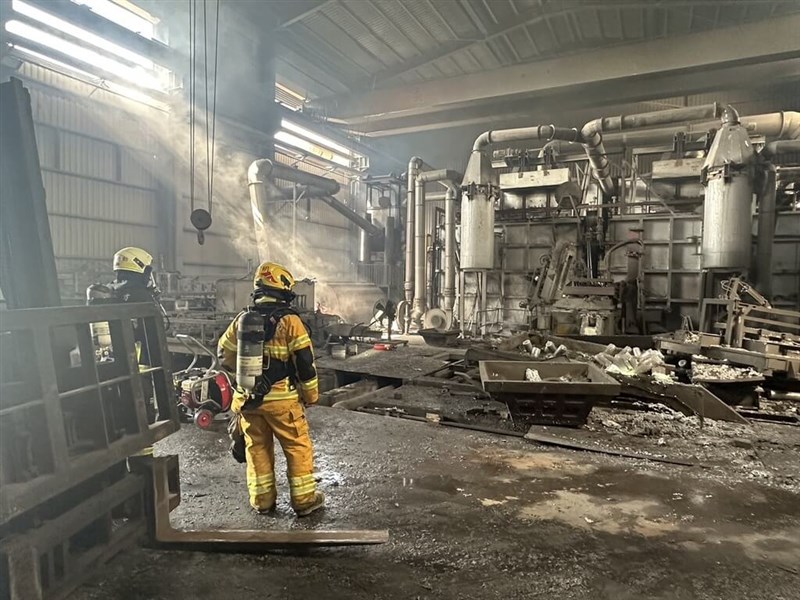In this highly detailed and well-lit photograph, we find ourselves in a slightly wider-than-tall industrial setting, showcasing the aftermath of an intense fire. The scene is dominated by two firefighters, positioned on the left side of the frame and dressed in full firefighting gear, featuring vivid yellow suits with reflective yellow stripes and oxygen tanks secured by black harnesses. The firefighter on the right is fully visible, while the other is partially obscured but identifiable by their helmeted head and equipment. The industrial environment is marked by an array of tanks, tubes, and piping visible in the background on the right. The floor is covered in debris, reminiscent of ashes, broken equipment, and possibly even water, suggesting recent firefighting efforts. The factory-like space is bathed in natural light streaming in from horizontal windows on the upper left, casting beams of light that pierce through lingering smoke, illuminating the devastation below. Amid the wreckage, a small red machine with a red wheel stands out, nestled between the two firefighters, adding a splash of color to the otherwise gray and smoky setting.